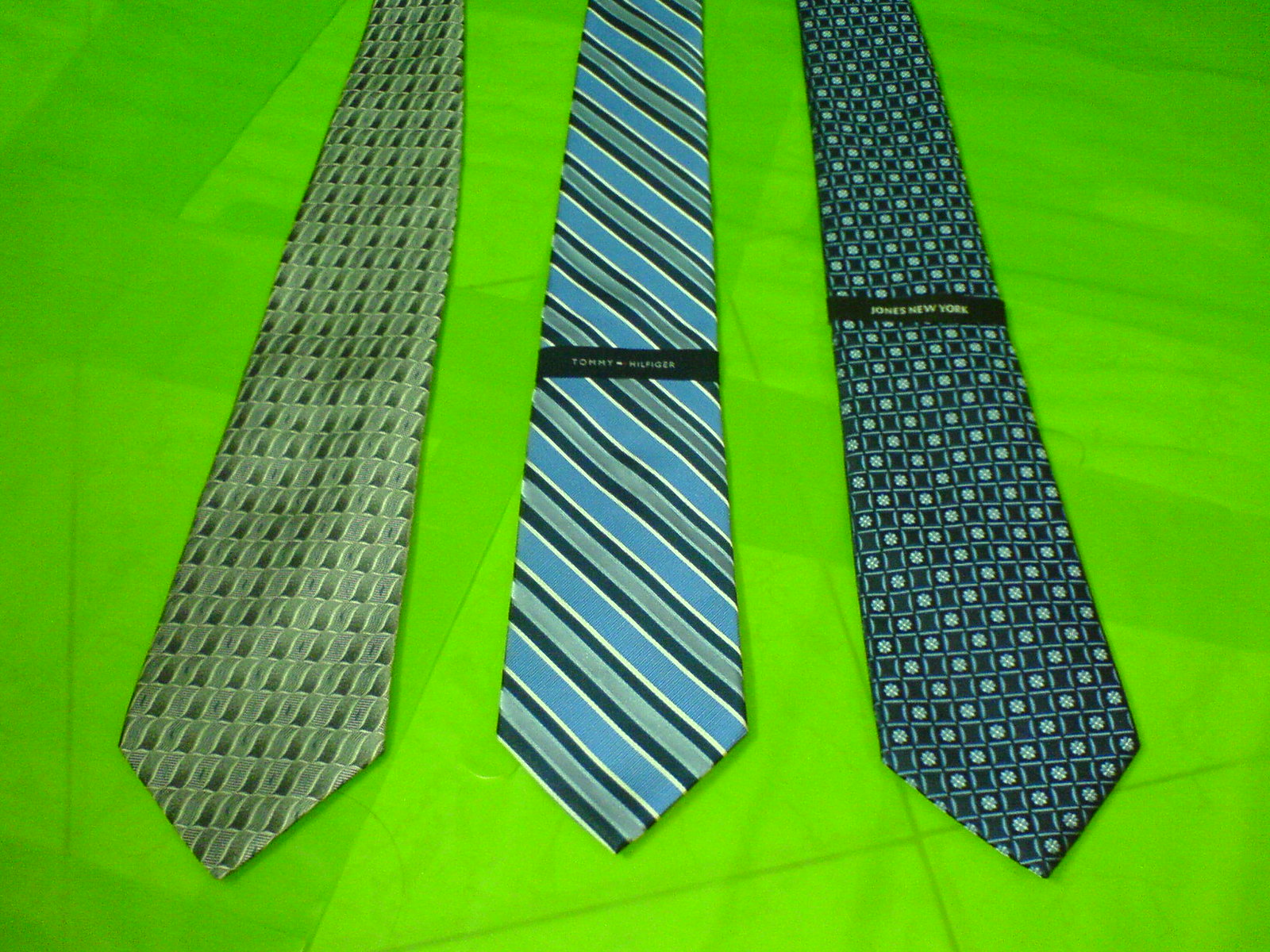This detailed photograph captures an assortment of three ties laid flat across a green-tiled background. The ties are positioned from left to right and only the wider, pointed ends are visible. The tie on the left is a grayish tone, adorned with a pattern of dark gray rectangles. The middle tie, identified as a Tommy Hilfiger, showcases alternating blue and gray stripes angled from left to right. On the right, a dark blue Jones New York tie features a square pattern with varying shades from dark blue to white squares interspersed with dots. The background, a solid green, appears to be composed of tiled squares, adding a contrasting texture to the elegant arrangement of the ties.